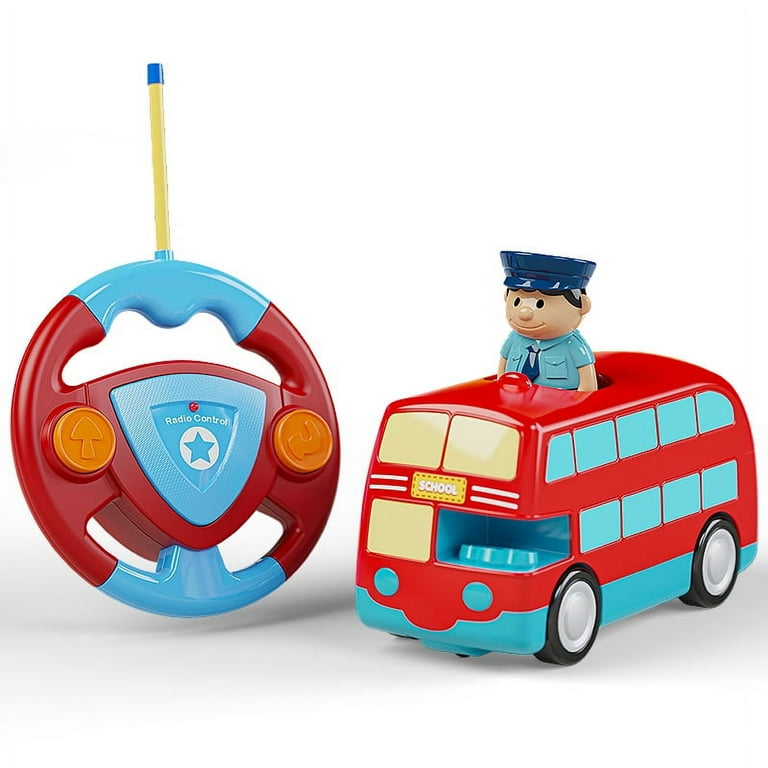This image features a vibrant, playful remote-control double-decker school bus toy designed for young children. The bus, predominantly red with blue accents, has charmingly exaggerated features, such as blue-tinted windows and black-and-silver wheels. Its front includes yellow windows, headlights with an eye-like appearance, and "school" written across the side. Atop the bus, a friendly, cartoonish bus driver figurine sticks out. He sports a blue police-like hat, a light blue shirt with double pockets, a dark blue tie, and a cheerful expression.

Accompanying the bus, on the left side of the image, is its round, steering wheel-shaped remote control. The vividly colored remote features red and blue sections, two orange buttons (one with an upward arrow and the other with a left-turn arrow), a blue triangle emblazoned with "Radio Control," and a small star at the center. An antenna extends from the remote, reflecting its interactive and fun nature for young users. The toys are displayed against a clean, white background with a faintly gray floor, giving the entire setup a polished, advertisement-ready appearance.